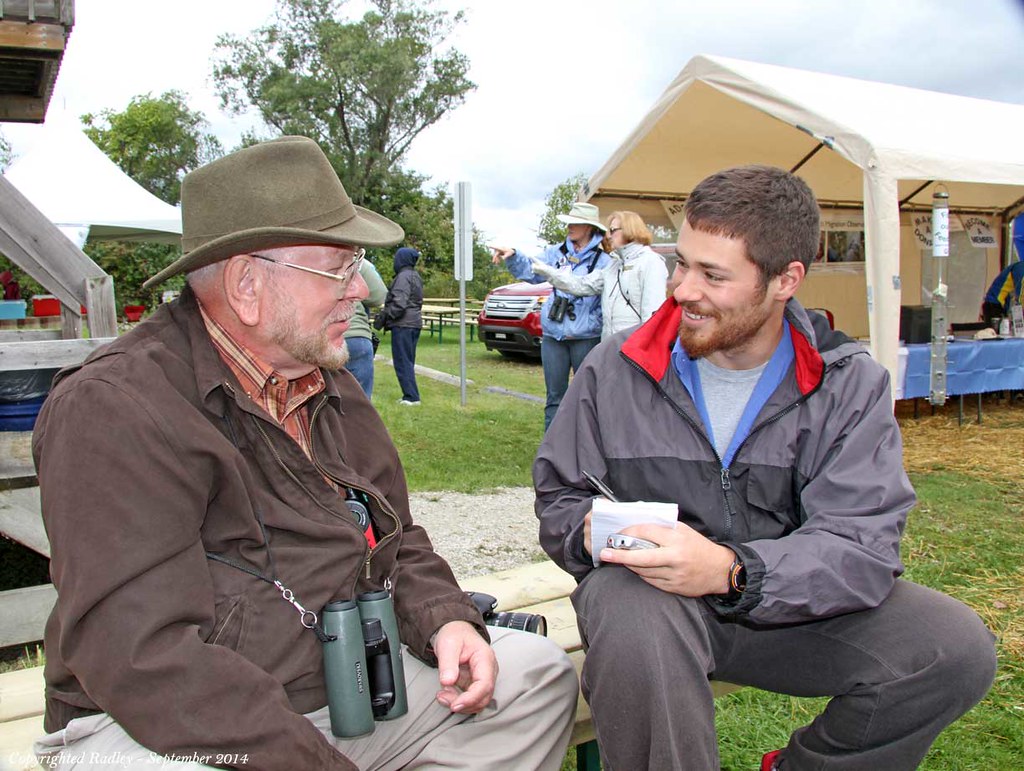In this photograph, two men are seated on a wooden bench, seemingly engaged in a discussion. On the left is an older white male, likely in his 60s, who sports a greenish-gray brimmed hat and gold-rimmed glasses. He has a short gray beard and mustache, and his attire includes a brown plaid button-down shirt under a brown jacket, khaki pants, and a pair of green binoculars hanging around his neck. Beside him on the bench rests a black DSLR camera.

Next to him, on the right, is a younger white male, approximately 29 years old, with short brown hair and a thick reddish-brown beard and mustache. He is dressed in a light gray t-shirt layered with a multicolored windbreaker featuring gray, blue, and red hues. He wears gray jeans and holds a pen and pad, as if interviewing the older man, listening and smiling attentively.

The background suggests they are at a festival or outdoor event, with numerous booths covered by white canopies, a grassy area, and people dressed in windbreakers and puff coats. A red pickup truck and other vehicles can be seen in a nearby parking lot, and the scene is framed by an array of trees and an overcast sky.